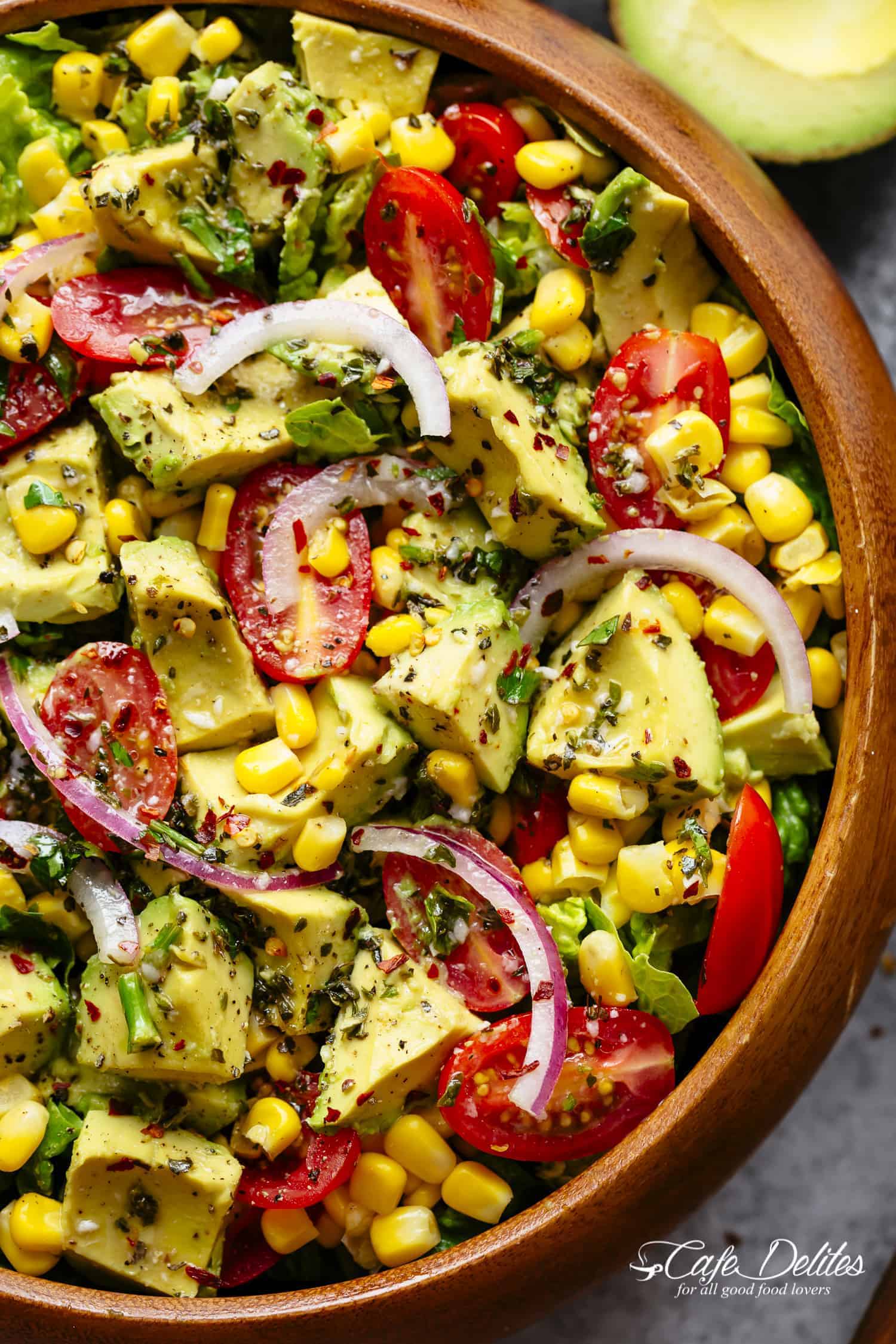The image showcases a vibrant and appetizing mixed salad in a wooden bowl taking up most of the screen. The salad features a variety of colorful, fresh vegetables including chopped avocado, sun-dried or grape tomatoes cut in half, red onions, and small pieces of corn, all mixed together and generously seasoned, possibly with olive oil. Notably, there's an uncut piece of avocado on the top right of the salad. This culinary delight rests on a marble or gray granite table, providing an elegant backdrop. At the bottom right of the image, the words "Cafe Delites: For All Good Food Lovers" are prominently displayed, highlighting the delightful and healthy appeal of this beautifully arranged dish.